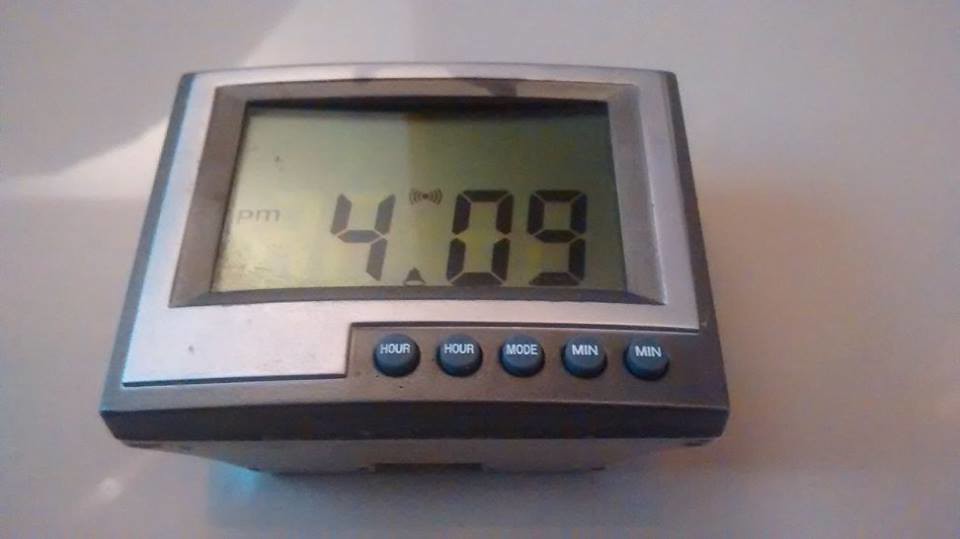In this color photograph, a small, square digital clock is prominently featured, centered against a white background that appears to be a white table or surface. The clock displays the time 4:09, which could be either a.m. or p.m., as it's not specified in the photograph. The clock itself is surrounded by a silver stainless steel outline and a gray outer edge, which could be either hard plastic or metal. The display area consists of a green digital screen framed twice: once by a black inner frame close to the display and then by a lighter silver frame. Below the screen, there are five round buttons arranged in a row; these are labeled in white with functions such as "hour," "mode," "minute," and "minute." 

An intricate play of light and shadows is present; curved sunlight is hitting the clock from the left-hand side, casting slightly bluish shadows towards the bottom left and an orangey shadow to the right. The digital screen itself shows some unreadable small text on the left side, in addition to the clear "4:09" time in a black display. This detailed view of the clock suggests not only a functional design but also aesthetic elements highlighted by the ambient lighting and shadows in the photograph.